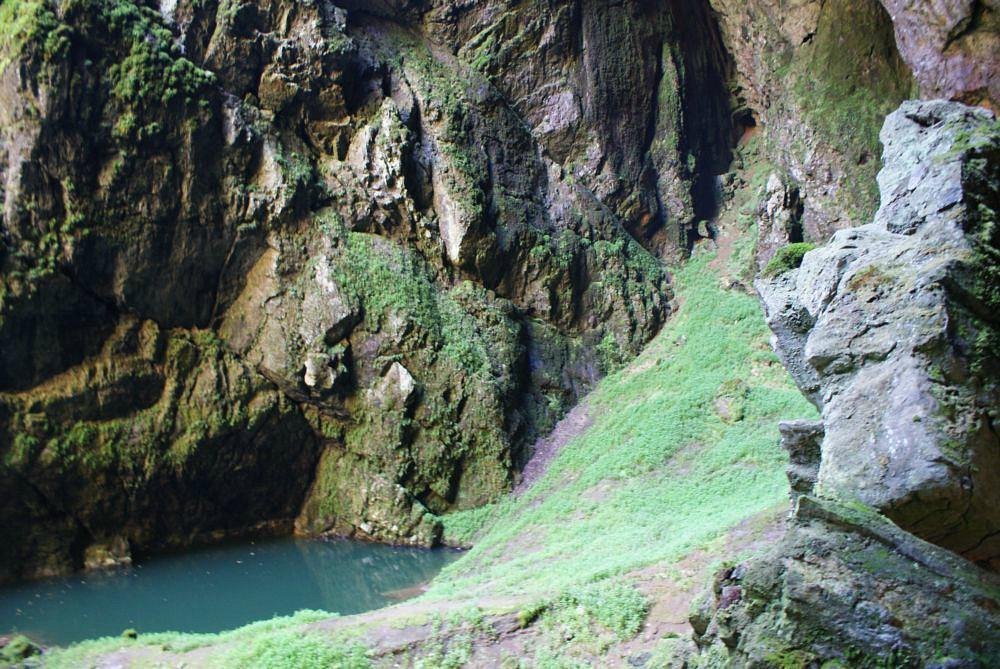The photograph captures a secluded grotto nestled within the crook of a large mountain or cliffside. Dominating the scene are rocky surfaces in the top right, top left, and bottom right corners, with hues of gray and white, marked by jagged, broken rocks. These rocky areas are lushly adorned with short green, moss-like grass, extending to the moss-covered cliffside visible on the top left. In stark contrast, the bottom left corner features a very dark blue, stagnant pool of water dotted with white bubbles. The rocks encircling this pool appear slightly more brown and damp compared to the others. The overall colors in the image are a natural blend of gray, green, blue, and hints of brown. The scene exudes a sense of isolation, with no presence of people or text in the image. The water’s murky blue adds to the mysterious, undisturbed aura of this hidden grotto.